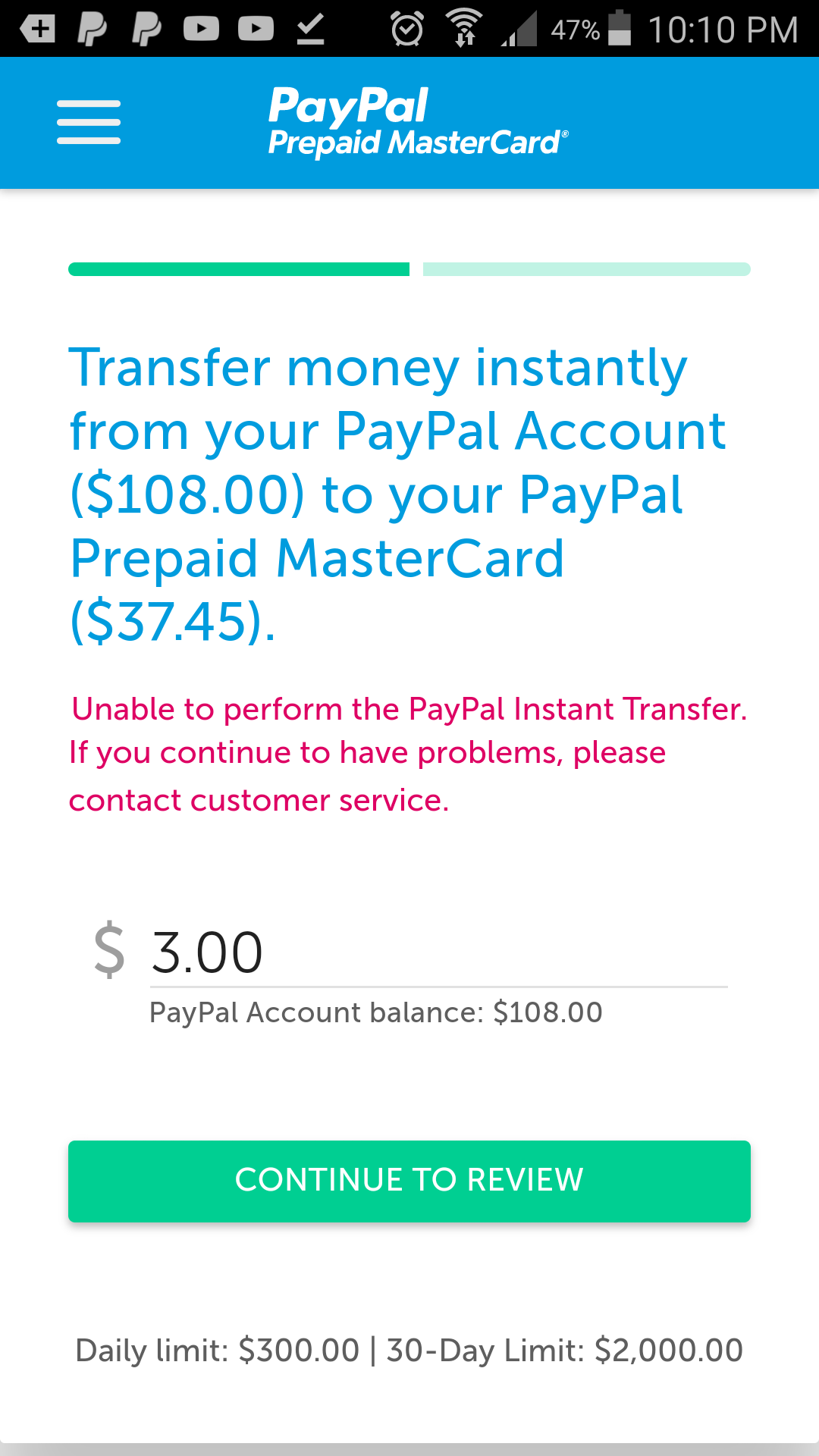The screenshot captures a detailed snapshot of a mobile phone screen. At the very top, a black notification bar displays gray icons. The sequence includes a banner with a black plus sign, a double "P" icon repeated twice in gray, two gray boxes with a black triangle, and a gray checkmark with an underline. A small clock icon appears next, followed by a volume control icon with gray arrows pointing up and down below it. The signal strength is shown with two bars, and the battery icon is outlined and filled to indicate 47% charge. The time displayed is 10:10 PM.

Below the notification bar, the screen transitions to a turquoise blue section. On the left are three white horizontal menu bars, next to the large white text "PayPal" followed by "prepaid MasterCard." 

Beneath the turquoise section, the background turns white, segmented by one medium green and one light green line. Below, bold blue text states, "Transfer money instantly from your PayPal account ($108) to your PayPal prepaid MasterCard ($37.45)." Following this is a pink message reading, "Unable to perform the PayPal instant transfer. If you continue to have problems, please contact customer service." 

Further down, a gray dollar sign icon is followed by "$3.00" in black text, which is separated by a fine gray line. Next, "PayPal account balance: $108" is displayed. Beneath this, a green banner spans the screen width, reading "Continue to review" in white text. Below the green banner, smaller text states "Daily limit: $300 / 30-day limit: $2,000," ending with a thick gray line.